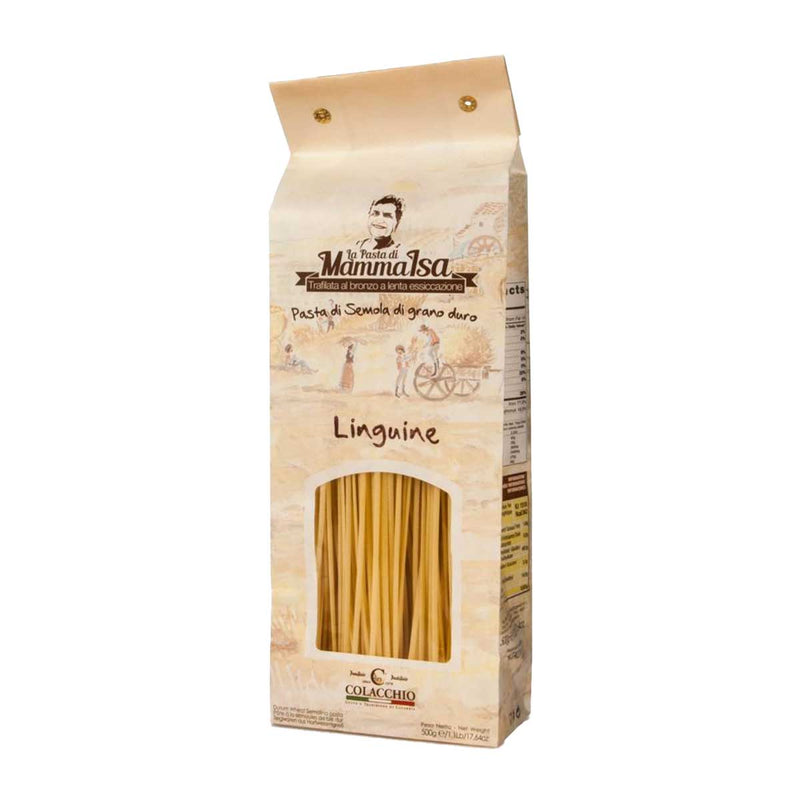This image shows a tall, tan-colored package of linguine pasta characterized by a detailed, artistic rendering. The main design includes a nostalgic, washed-out illustration of a rural scene: a house with a water wheel forms the backdrop, while the foreground features various characters - a woman standing, a wagon loaded with hay, one person taking hay from the wagon, another handing it down, and additional figures including one reclining on the left. The bottom half of this scene depicts an expansive hay field.

Prominently featured at the top of the package is the logo "La Pasta di Mama Isa," illustrated with a broadly smiling woman with short dark hair. Just below this logo is some additional Italian text in white against a brown banner. Below the banner, "Pasta di Semola di Grano Duro" is written, followed by "Linguine" under the wagon illustration. 

An open window in the lower half of the package reveals the actual linguine noodles inside. Near the bottom of the package, there’s a logo that reads "Colacchio," flanked by a tricolor strip in the colors of the Italian flag – green, white, and red. On the right side, partially seen due to the angle, are white and yellow nutritional facts boxes positioned one above the other. The package material appears to be paper with metallic rivets towards the top providing a rustic finish.